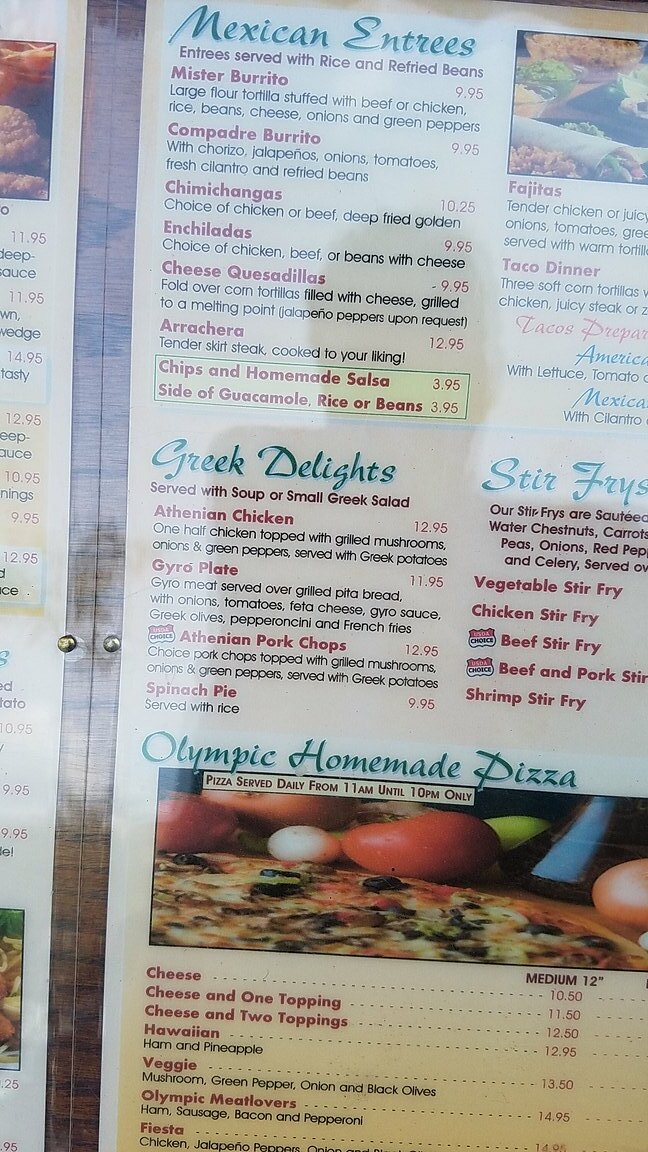This is a photograph capturing the menu of an international-style restaurant, positioned slightly askew towards the right. The menu is folded in the center, revealing a clear plastic cover along the fold, through which a brown tabletop is visible. Two small gold-colored fasteners are positioned in the center of the plastic covering. The menu features a diverse range of items including Mexican entrees, Greek delights, stir-fries, and Olympic homemade pizza. Near the bottom of the page, there's a rectangular photograph showcasing a side view of a pizza adorned with vegetables in the background. At the top right of the page, about half of a photo depicting burritos, rice, and condiments can be seen. A subtle shadow, possibly of a person's head and shoulders, is reflected on the menu's surface, adding a human touch to the scene.